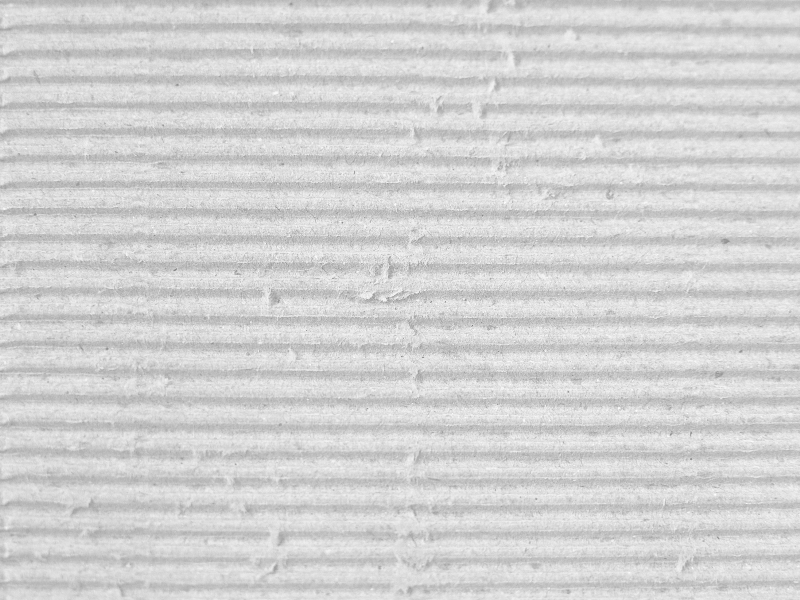This horizontal, slightly rectangular, up-close photograph captures a detailed view of what appears to be an air filter, exhibiting a textured and layered appearance. The filter has prominent white horizontal lines interspersed with gray ones, indicative of collected dirt and debris. The white parts are raised, possibly highlighting trapped particles. Despite initial impressions of it resembling a textured paper towel due to its slightly crushed parts and raised channels, the gray hues and spots suggest it is dirty, reinforcing the idea that it is an air filter. The material's subtle puckering pattern adds a plaster-like, layered ambiance, detailed with small dots and a heavy texture, emphasizing its purpose in filtration.